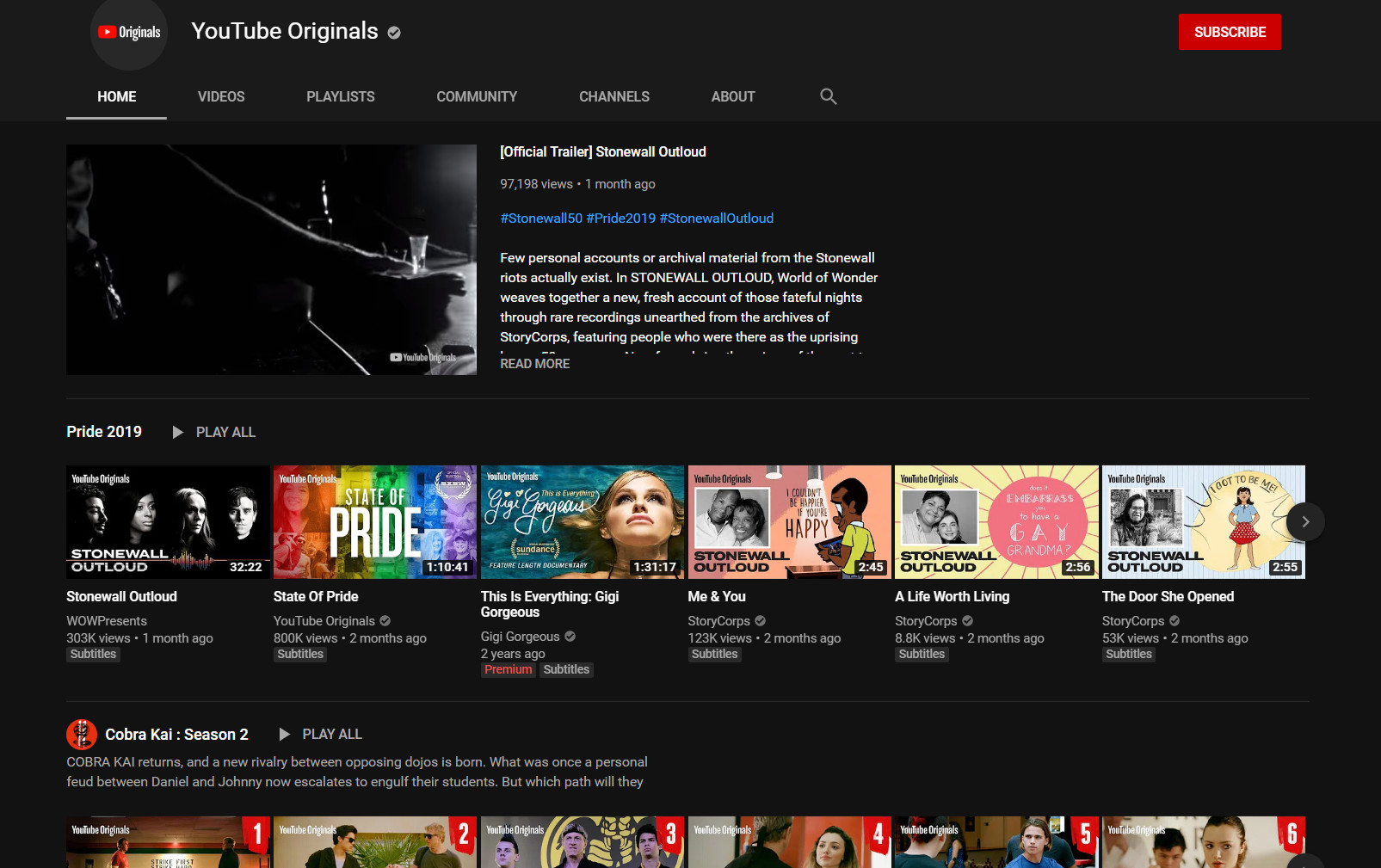This is a detailed screenshot of the YouTube Originals channel. The background color is black, with "YouTube Originals" prominently displayed, accompanied by a verified checkmark. To the right, there is a red "Subscribe" button. Below this header is a menu bar that includes options like Home, Videos, Playlists, Community, Channels, and About, along with a search bar. The Home tab is currently selected.

The first featured video is an official trailer for "Stonewall Outloud," boasting 97,198 views and posted one month ago. The trailer’s thumbnail is in black and white, and a brief description lies underneath.

Beneath this, there is a section titled "Pride 2019," featuring a "Play All" option. This section showcases various videos related to Pride 2019, arranged in a row. The videos are:

1. "Stonewall Outloud"
2. "State of Pride"
3. "This Is Everything: Gigi Gorgeous" (also tagged with YouTube Premium)
4. "Me and You"
5. "A Life Worth Living"
6. "The Door She Opened"

Each video includes a "Subscribe" tag and lists details such as the upload date, the uploader’s name, and the number of views. 

The subsequent section is titled "Cobra Kai Season 2," also featuring a "Play All" button. It contains six videos from the series, placed in a sequence.